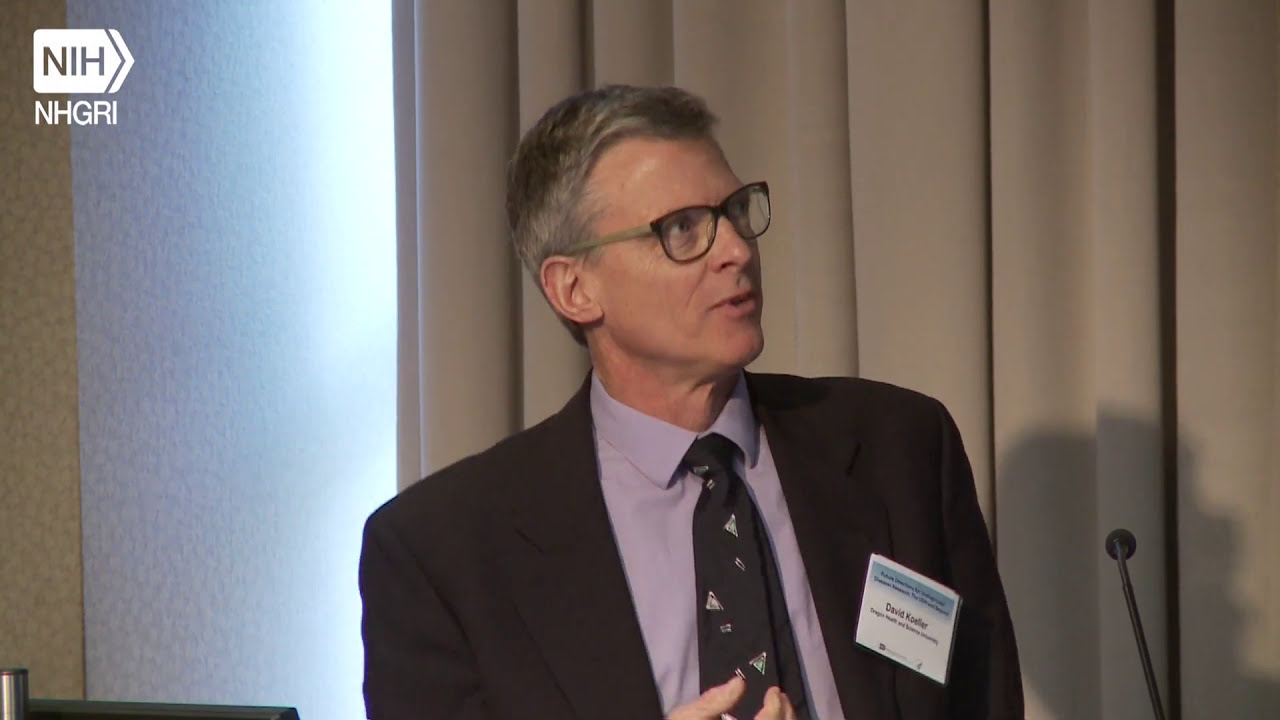The image displays a middle-aged Caucasian man, likely in his late 40s or early 50s, standing against a backdrop of a white wall and beige pleated curtains. He is dressed in a black suit with a light-colored collared shirt (gray or blue) and a dark tie featuring a small white triangular pattern. The man has short, grayish-brown hair and wears black-framed glasses. Attached to the left side of his suit jacket is a name tag with a blue top section and white bottom, inscribed with his name, possibly "David Kohler" or "David Keller." He appears to be at a press conference or giving a lecture, indicated by his lip position as if mid-speech and his right hand slightly raised with the thumb and two fingers visible. On the bottom right of the image is a slim, small microphone directed towards him. In the top left corner, the symbols NIH and NHGRI are prominently displayed.